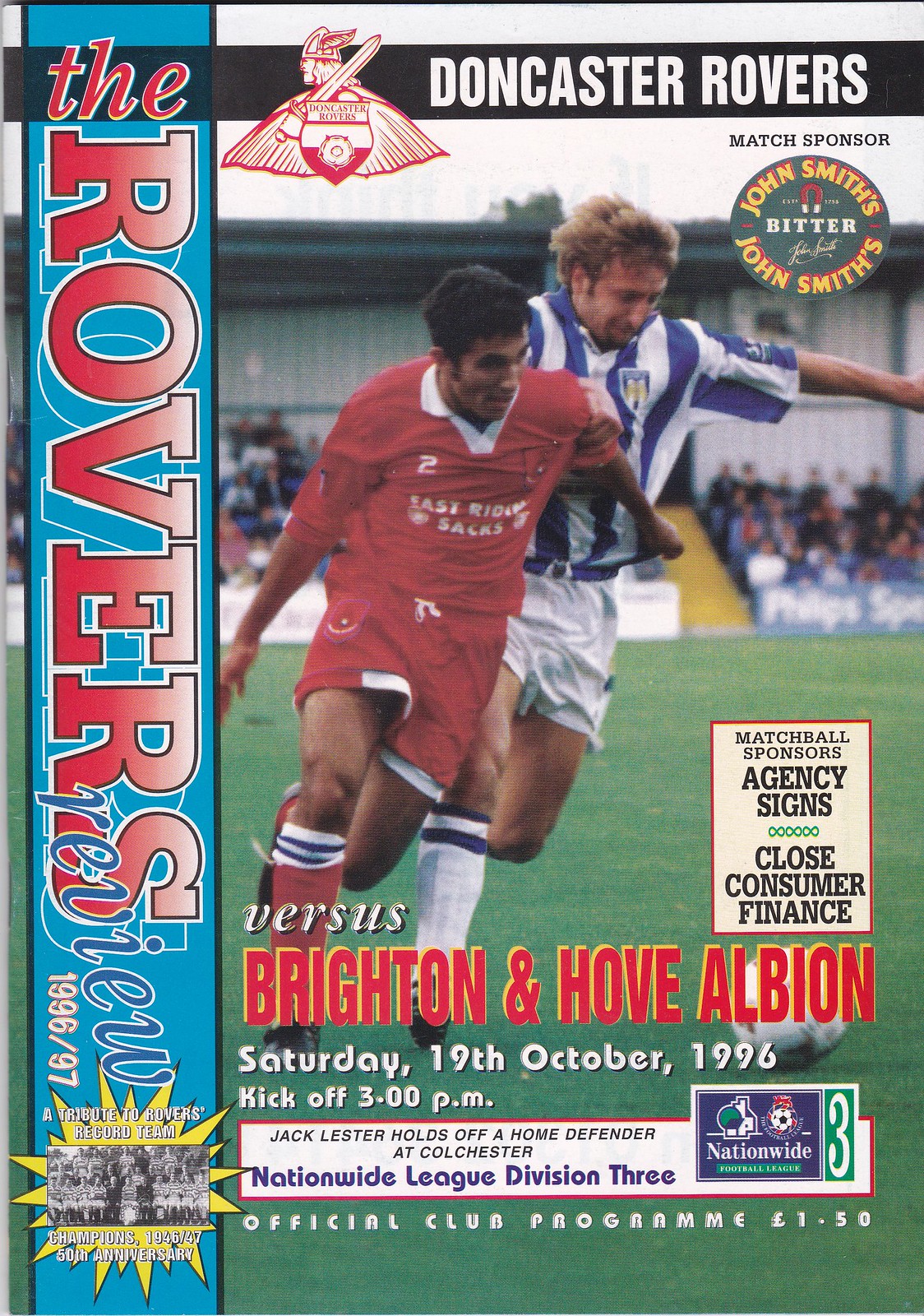The image is a detailed scan of a soccer magazine cover, titled "The Rovers Review," which showcases an action-packed photograph from a match between Doncaster Rovers and Brighton. The cover prominently features two players vigorously competing for the ball—one donning a red uniform and the other in a white uniform with blue stripes. The backdrop displays a blurred crowd of spectators and green turf, indicative of a small soccer stadium. The colors have a slightly faded 90s-era appearance but remain vivid. 

At the top of the cover, a dark band bears the text "The Doncaster Rovers" alongside the club’s emblem, depicting a Viking with a winged helmet, a sword on its shoulder, and a shield inscribed with "Doncaster Rovers." Additionally, the match sponsor's name appears underneath. The left side of the cover features a vertical blue band with "The Rovers Review" written in bold red text from top to bottom. The date is highlighted as Saturday, 19th October 1996, marking the issue as an official club program for a Nationwide League Division 3 match. The caption below the image notes Jack Lester holding off a home defender at Colchester, adding context to the dynamic scene displayed.